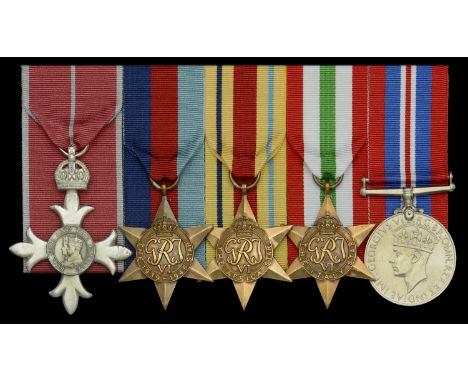The image features five distinct medals against a black background. Starting from the left, the first medal is attached to a red fabric ribbon and consists of a silver cross-like structure adorned with a silver crown at the top. Below the crown, there is a circular silver cone embellished with four silver floral patterns around it. The second medal, along with the third and fourth, has a six-pointed star design. These three stars are made of bronze and feature the letters GRJE engraved in the center. Each star is attached to a different colored ribbon: red, dark blue, light blue, yellow with blue and red stripes, and green with white and red stripes. Finally, the fifth medal on the far right has a red, white, and blue fabric ribbon and showcases a large silver coin depicting the side profile of a crowned king facing left, with some legible inscription around it, including possibly the word "George." The medals are captured in a well-lit and clear setting, highlighting the intricate details and varying ribbon colors.